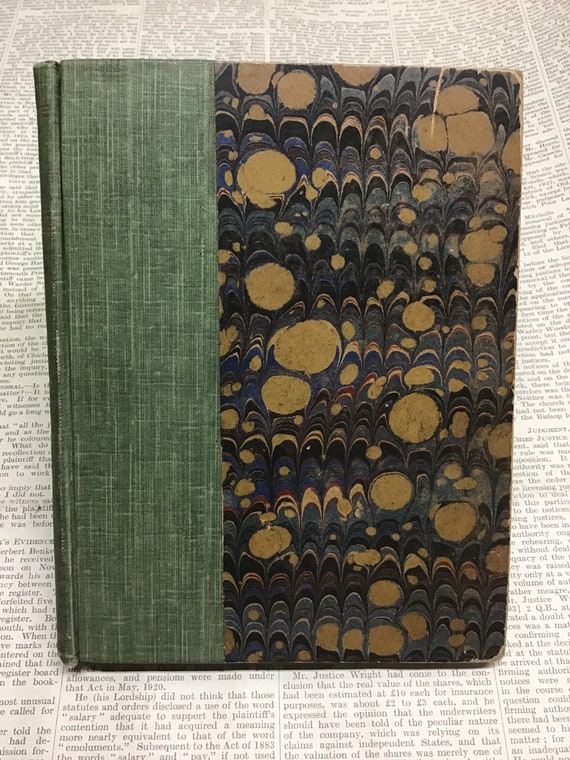This color photograph features a visually striking hardbound book resting atop what appears to be a large sheet of newspaper or a page from a grand book, characterized by small black type font arranged in columns. The book itself boasts an intricate and elegant design. Its spine and the left side of the front cover are adorned with a textured green linen material, possibly striped or carrying visible marks suggestive of prior bending. The remaining portion of the front cover is enveloped in a stunning marbled paper, vividly decorated with an array of colors including purples, golds, blacks, and reddish hues, as well as browns and blues forming a swirling, inkblot-like pattern of waves and circles. This combination of the green linen and the colorful marbled paper creates a captivating visual contrast, making the book a beautiful display of old-world craftsmanship.